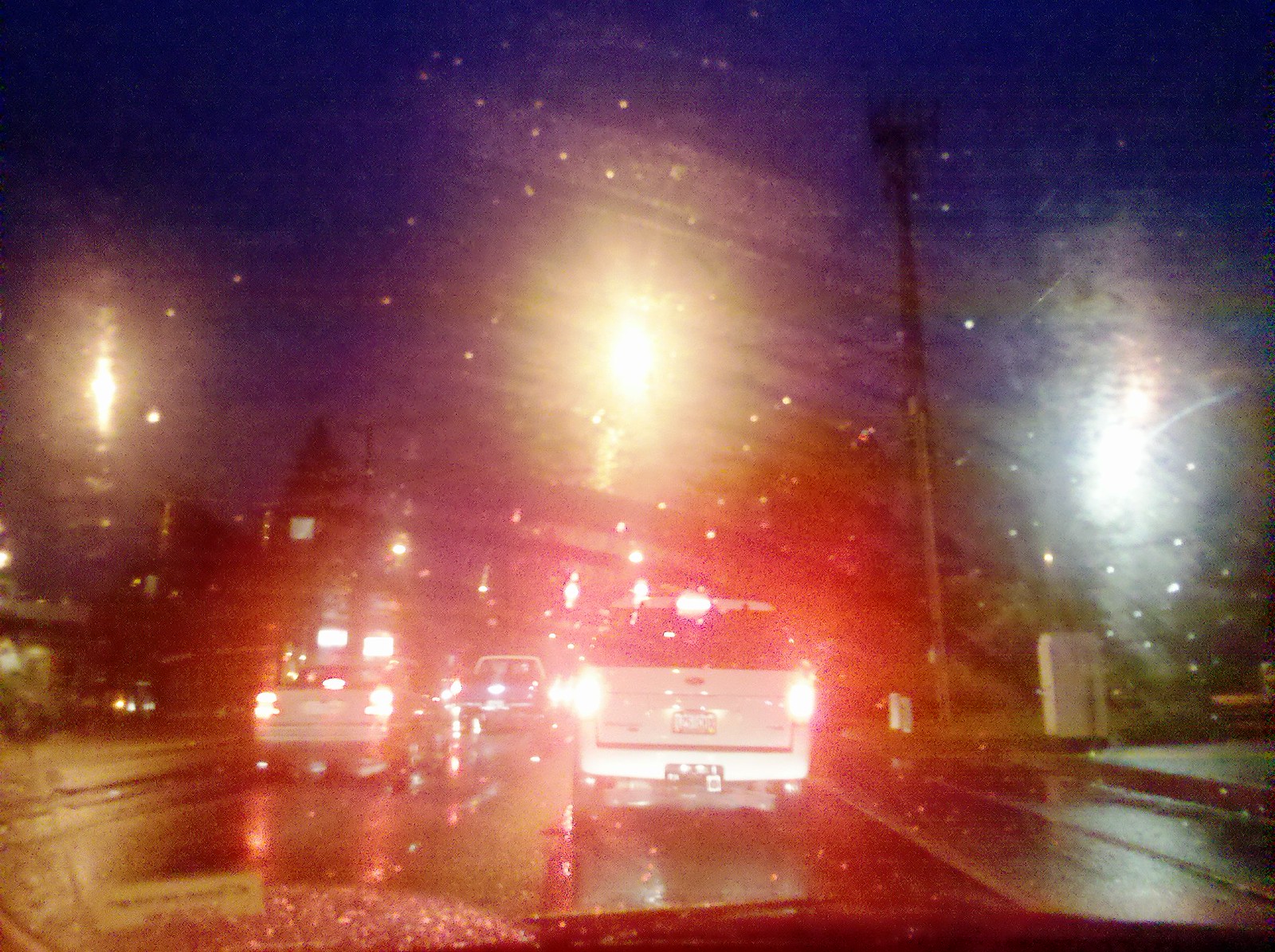This captivating composite photograph blends several distinct images to create a vivid and artistic scene. The base layer features a typical urban road with a few cars navigating under a streetlight, highlighting regular traffic flow. Adding to the surreal quality, each vehicle is enveloped in a red filter or glow, casting an otherworldly ambiance over the scene. Enhancing this, the upper layers of the composition introduce an array of luminous elements that resemble pyrotechnics. A multitude of glowing lights, predominantly amber and silver-hued, burst across the top of the image like sparkling fireworks. The combination of dynamic traffic imagery with glittering special effects creates a visually striking and multi-layered depiction of an ordinary city moment transformed into an extraordinary visual spectacle.